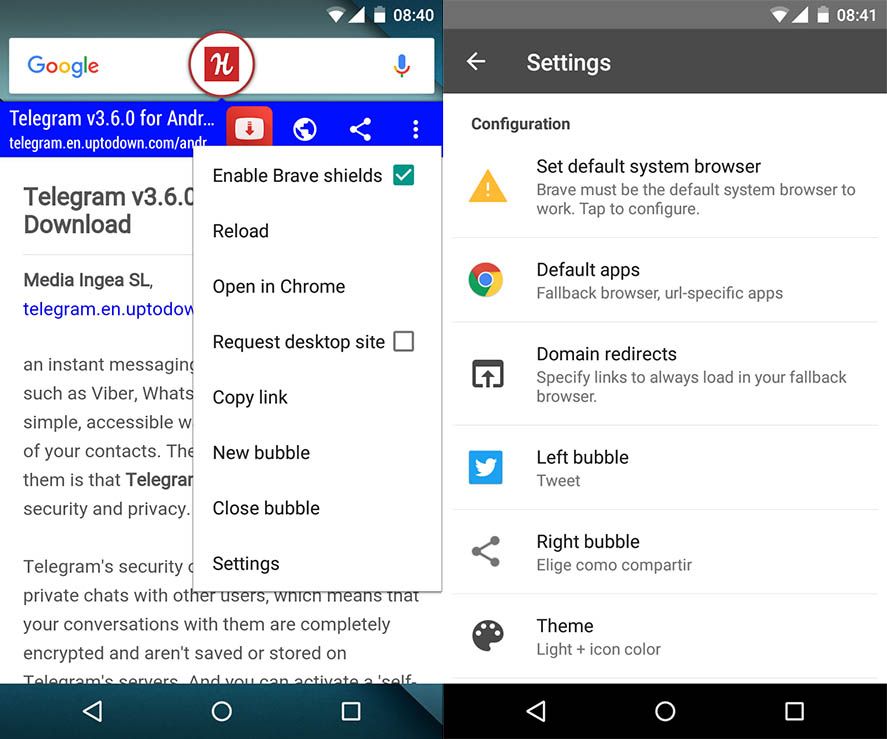The image shows two screenshots of a cell phone interface side by side. The left screenshot features a green status bar at the top, displaying cellular signal bars, Wi-Fi signal strength, a battery icon, and the time reading "8:40." Below the status bar is a Google search bar, followed by text indicating "Telegram v3.6.0 for Android, Telegram download". A pop-up window is visible, displaying options such as "Enable Brave Shields," "Reload," "Open in Chrome," "Request desktop site," "Copy link," "New bubble," and "Close bubble."

The right screenshot, with a gray status bar at the top and the time "8:41," shows a settings menu. At the top, a left arrow is followed by the text "Settings." The menu items include "Configuration," "Set default system browser," and a note indicating "Brave must be the default system browser to work. Tap to configure." Further down are additional settings labeled "Default apps," "Fallback browser," "URI specific apps," and "Domain redirects," with a note: "Specify links to always load in your fallback browser." At the bottom, it has icons for "Left bubble, tweet" and "Right bubble, eligible," with some text in Spanish "elige, como, compare." The menu also references "Light plus icon color," suggesting that the right screenshot is part of the Brave browser configuration process following its download.